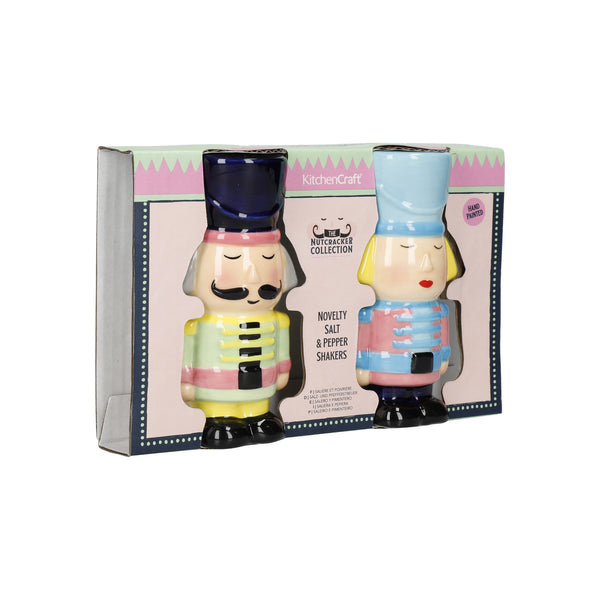This image features two Nutcracker-themed salt and pepper shakers encased in a decorative box. The top of the box prominently displays "Kitchen Craft" in white letters on a pink background. Below this, there are illustrated representations of two Nutcracker figures labeled as part of the Nutcracker Collection. These figures are depicted much like the actual shakers inside.

On the left is a male Nutcracker, distinguishable by his large black cap, a turned-up black handlebar mustache, a vest with yellow and pink stripes, and a black base. His pants are detailed with yellow and green hues. On the right stands a female Nutcracker, marked by her large blue cap, blonde hair, red lipstick, a pink and blue shirt, and blue pants with black shoes.

The box itself is adorned with blue borders and white dots, adding to its festive appearance. The nutcracker figures are carefully set in a way that they remain securely attached yet touchable within their packaging. This set of novelty salt and pepper shakers, part of the Nutcracker Collection, offers a whimsical holiday-themed addition by Kitchen Craft.